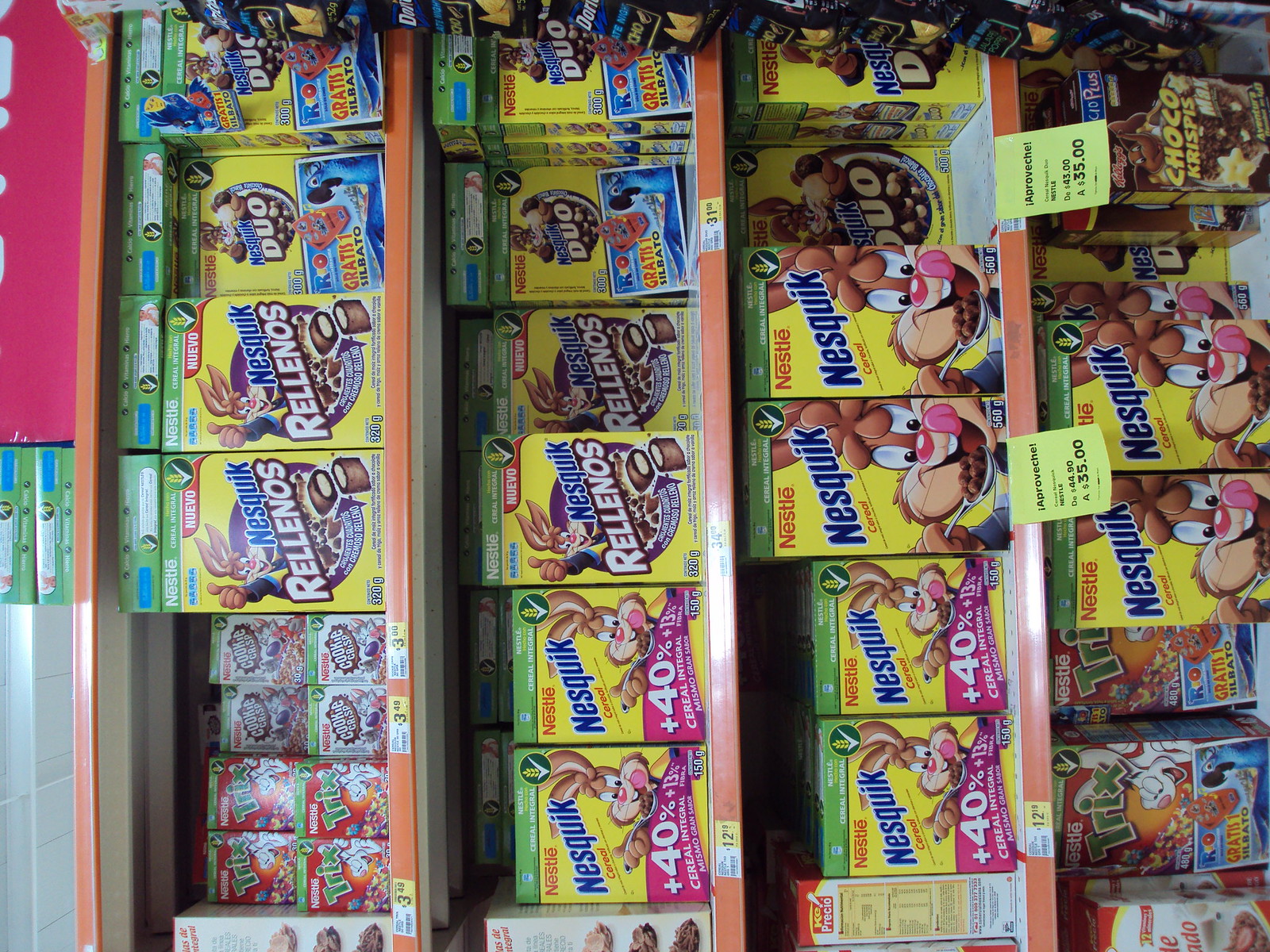In this image, which is oriented sideways, we see the aisle of a grocery store stocked with a wide variety of cereal options. Prominently displayed are multiple boxes of Nesquik cereal, featuring the iconic bunny mascot with its tongue out, eagerly poised to scoop some cereal. These Nesquik boxes come in different variations, some boasting "Plus 40%" and others labeled as "Rellenos," depicting pieces of cereal that are split open to showcase their fillings. Numerous price tags are visible, marked with "35.00" in what appears to be a foreign currency. In the upper left corner of the image, there are also boxes of Trix cereal and Cookie Crisp, along with an assortment of other cereal brands, all neatly stacked on the shelves. The overall atmosphere is that of a well-stocked store overseas with a colorful and diverse cereal selection.